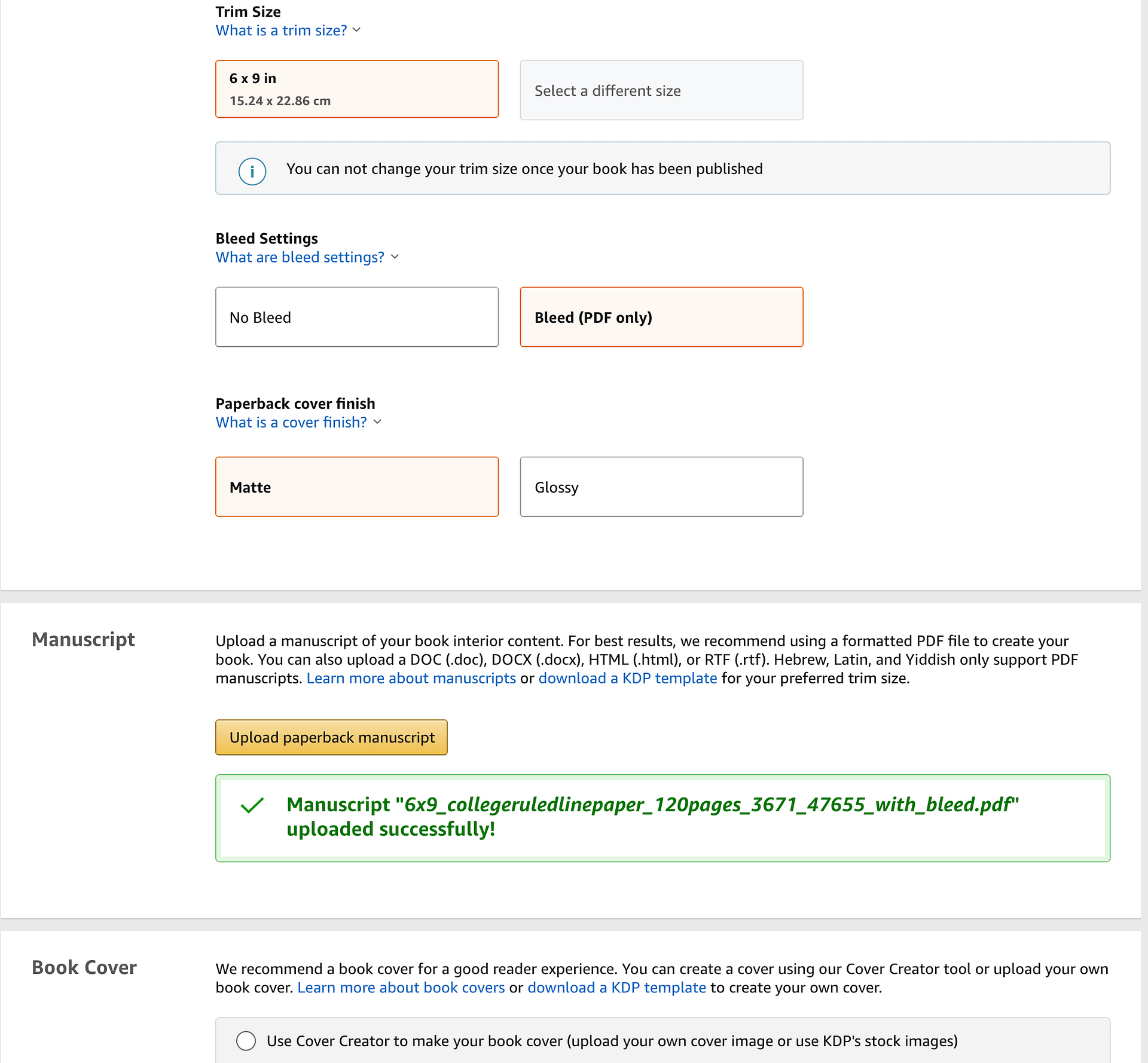The image features a variety of colored shapes and text on a white background, structured to explain different aspects of book formatting and settings:

1. **Trim Size Information:**
    - **Text in Black:** "Trim size" explained.
    - **Text in Blue:** Questioning "What is a trim size?"
    - **Orange Rectangle:** Contains the dimensions "6 x 9."

2. **Different Size Selection:**
    - **Gray Rectangle:** Indicates different size selections, including a blue circle with an eye icon, suggesting additional information available.

3. **Trim Size Note:**
    - **Gray Text Box:** States "You cannot change your trim size once your book has been published."

4. **Bleed Settings:**
    - **Text in Blue:** Questioning "What are bleed settings?"
    - **White Box:** Indicates "No Bleed."
    - **Red Rectangle:** Labeled "Bleed (PDF only)."

5. **Paperback Cover Finish:**
    - **Text in Blue:** Questioning "What is a cover finish?"
    - **Red Rectangle:** Marked "Matte."
    - **White Rectangle:** Marked "Glossy."

6. **Manuscript Information:**
    - **Text Box:** Contains information about the manuscript.
    - **Two Hyperlinks in Blue:** 
        - "Learn more about manuscripts."
        - "Download a KDP template for your preferred trim size."

7. **Upload Manuscript:**
    - **Yellow Rectangle:** Contains "Upload paperback manuscript."

8. **Manuscript Uploaded Confirmation:**
    - **Green Rectangle:** Has a green check mark stating "Manuscript."
    - **Text in Green:** Indicates a specific manuscript named "6 x 9_x"_ (underscored).

This detailed caption accurately provides a comprehensive description of the various elements displayed in the image.